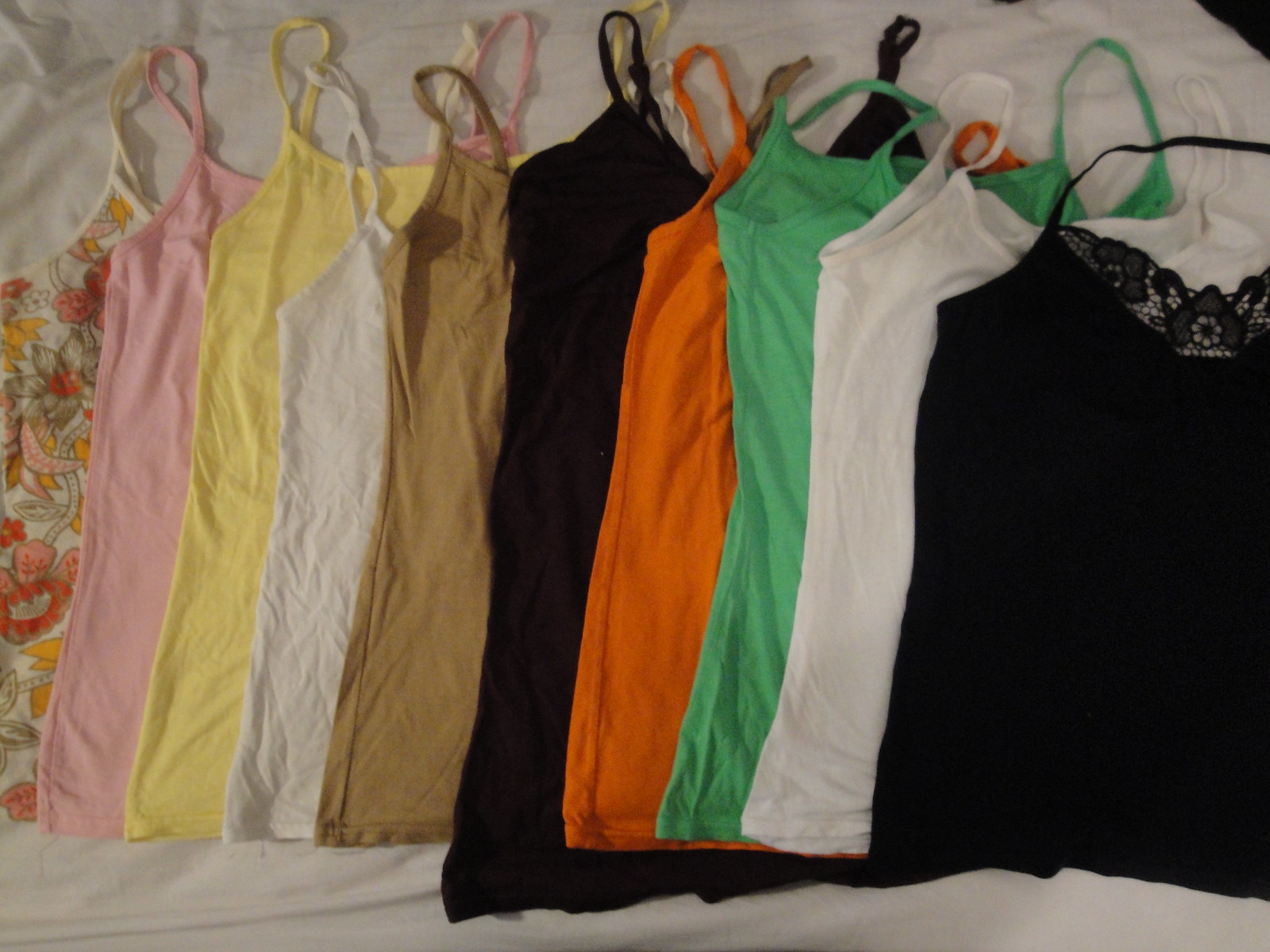The image features a collection of 10 camisoles neatly arranged on a white, slightly wrinkled sheet, which appears to cover a bed or mattress. In the upper right-hand corner, there's a small black triangle. The camisoles are spaghetti strap style and are laid out in a sequence from left to right. Starting on the left, the first camisole is a multicolored floral design with hues of orange, yellow, green, pink, and red, and it has a cream white near the string sleeves. Following this, the second camisole is a solid pink, the third is yellow, the fourth is white, the fifth is beige, the sixth is black, the seventh is orange, the eighth is green, the ninth is white again, and the tenth is black with lace detailing at the top. The camisoles, which vary slightly in size and shape, seem to be arranged with intention, as they are spread out slightly to display each one distinctly.